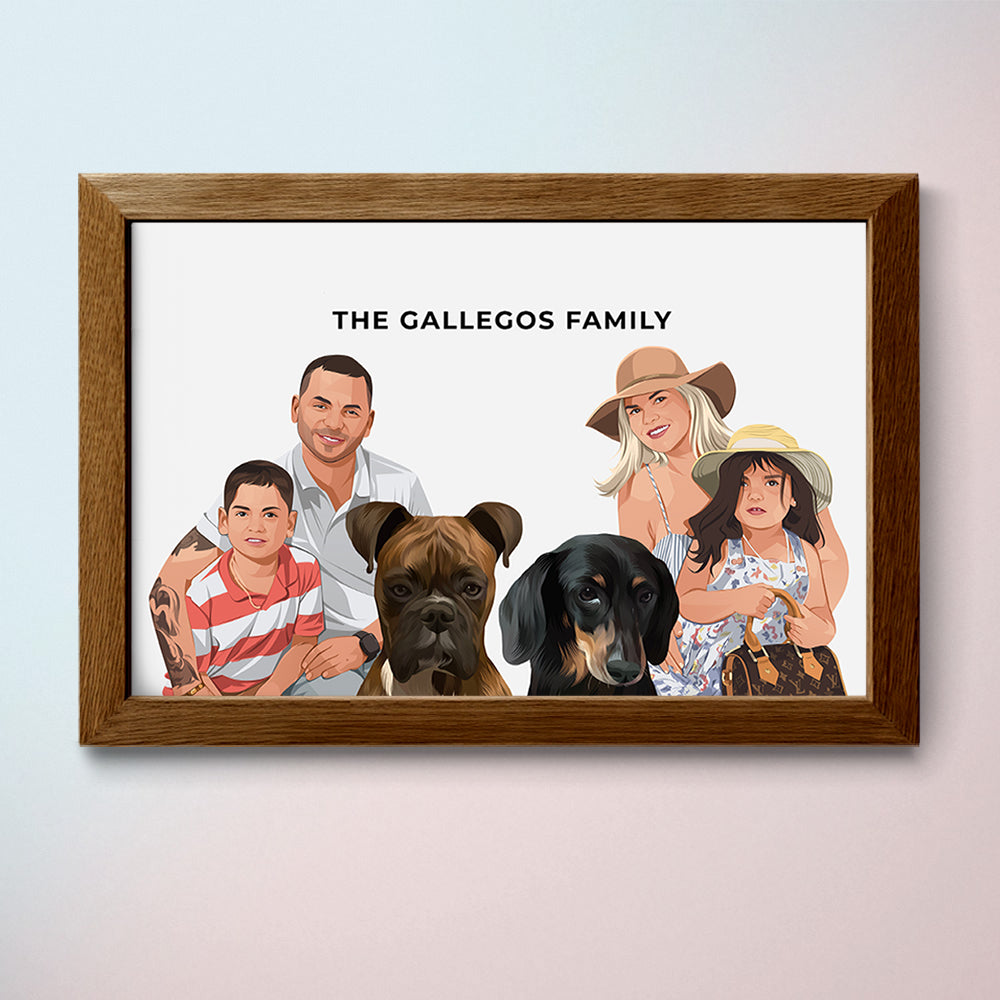The image is a cartoon-like, framed family portrait titled "The Gallegos Family," written in a sans-serif font. In the center, we see the father, who has a tan complexion and tattoos on his arm, holding a young boy dressed in a red and white horizontal striped shirt. Beside him stands the mother, a fair-skinned Caucasian woman with blonde hair, holding a young girl with brown hair. Both mother and daughter are wearing sundresses and hats. The young girl appears to love her purse, indicating it was likely given to her by her mom. In the foreground, two dogs are prominently featured as part of the family—a brown dog resembling a boxer, and a black dog.